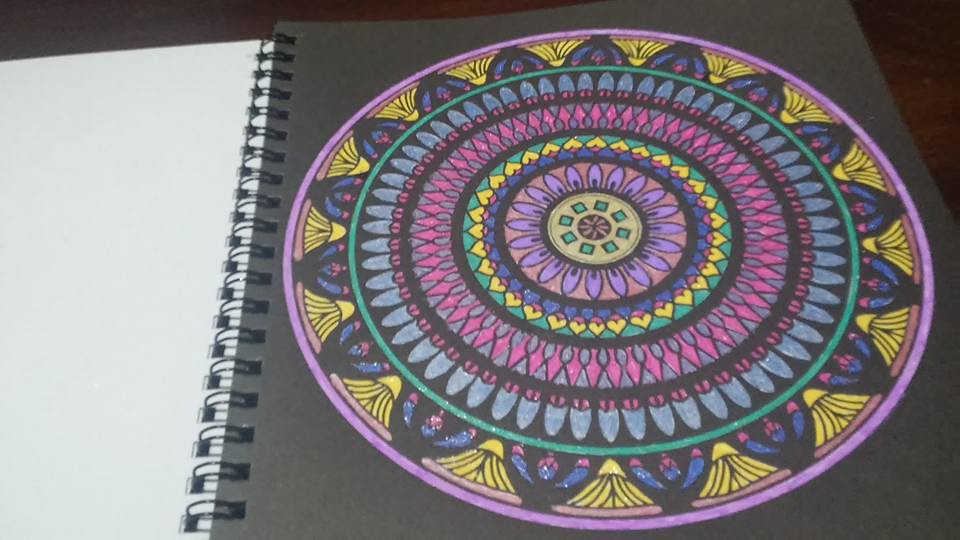The horizontally rectangular frame captures a spiral-bound art book viewed from a slightly downward angle. On the left side of the image, the black spiral binding of the notebook is visible, adjacent to a pristine white page. Dominating the right side of the frame is a striking piece of black art paper, prominently featuring a vivid, kaleidoscopic circular design. The outermost edge of the circle boasts a bright pink border, followed by a yellow scalloped pattern. Inside this, a green circular border encloses the central motif. The intricate kaleidoscopic effect is created by progressively smaller and more detailed concentric circles, each adding depth and complexity to the mesmerizing design.